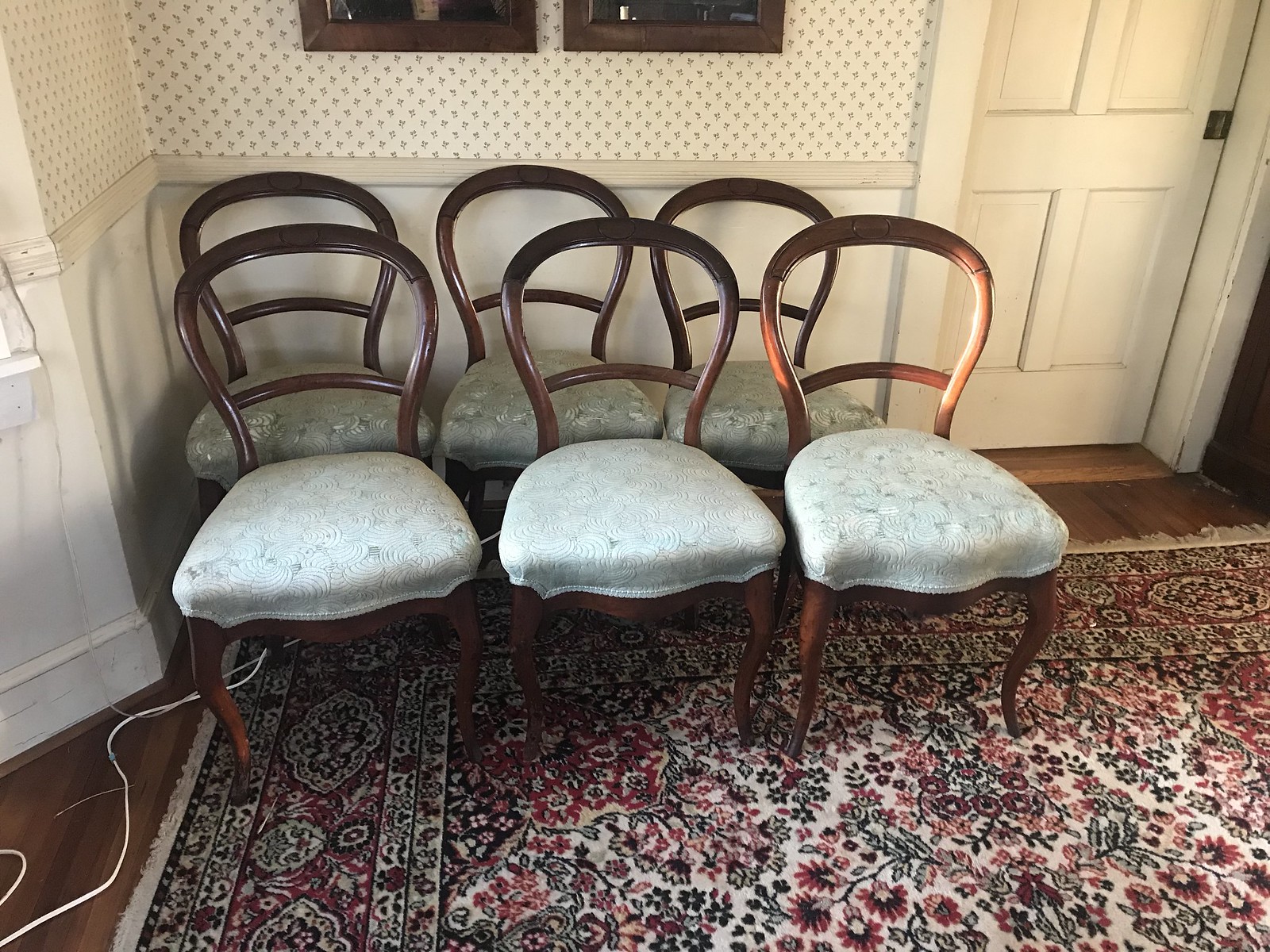The image depicts a bright, sunlit room, likely a dining area within a home. It is taken as a horizontally rectangular photograph, in realistic color. The background features a white wooden door on the right and a white wall with a white chair rail in the center and white wallpaper adorned with small floral designs above the trim. Below the chair rail, the wall is plain white. The wallpaper and paint create a quaint, cozy atmosphere.

The room's floor is made of brown hardwood planks, partially covered by a large, multi-colored area rug with intricate floral patterns dominated by reds, blacks, and accents of green. This oriental-style rug adds richness and warmth to the space.

Positioned prominently in the image are six matching wooden dining chairs set against the wall in two rows of three. The chairs feature dark brown rounded wooden backs and legs, with comfortable light teal to light gray cushions possibly made of velvet or a swirly fabric. The cushions are ingrained into the chairs' design, providing a soft, inviting seating area. Additionally, two mirrors with dark brown wooden frames are partially visible on the wall, adding depth to the room's décor.